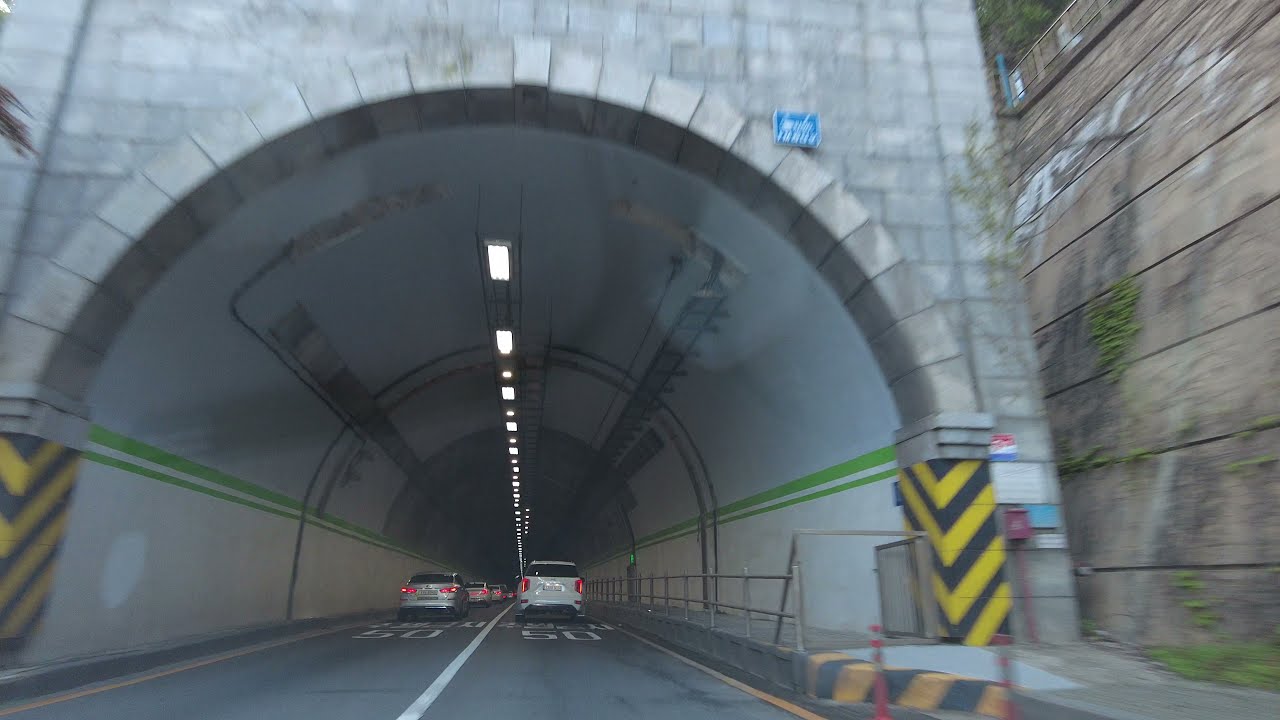The photograph captures the perspective of someone inside a car driving towards a tunnel on a multi-lane road. The car's windshield partially reflects, indicating the image is taken from the inside. The tunnel dominates the center of the image, framed by a round gray archway made of stone bricks. The entrance is marked with black and yellow safety stripes. On either side of the tunnel's entrance, a tan brick wall with patches of green ivy extends outward.

Inside the tunnel, which is rounded and appears to be made of smooth concrete, the lower part of the walls is painted a cream color adorned with green stripes, while the upper part is white. Illuminated lights hang down the center of the tunnel. Along the left inside edge, there's a raised sidewalk with a steel handrail, likely for maintenance workers. The walls are lined with painted arrows and the number 50, suggesting a speed limit. The roadway features a white line down the middle and yellow lines on the sides. Various cars are visible driving through the tunnel, under the bright daylight from outside.